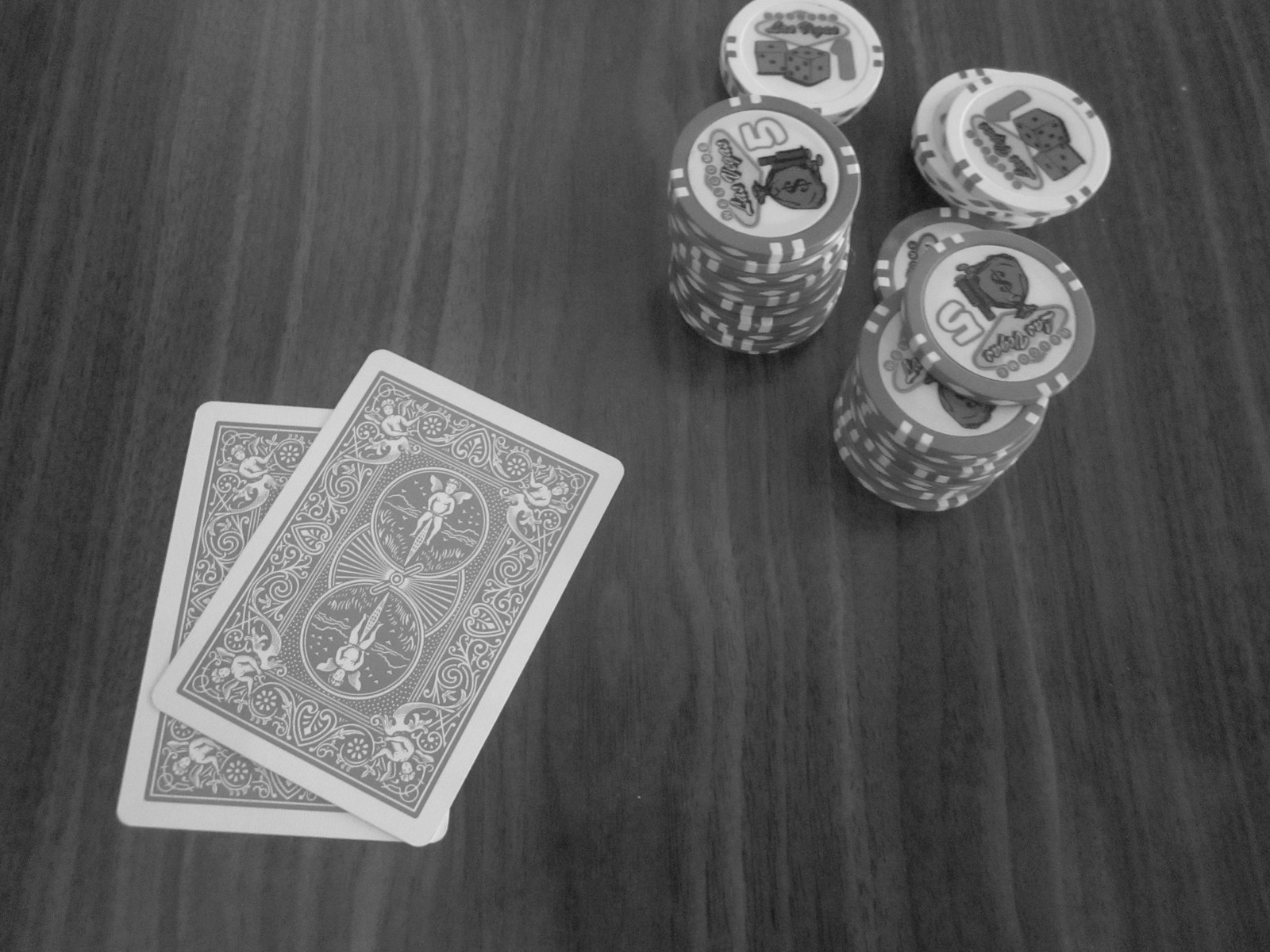In this black and white, landscape-oriented photograph, the rich, vertical wood grain of a table serves as the background. Near the lower left corner, two playing cards lie slightly askew, one atop the other at a slight angle to the right. These classic playing cards feature intricate borders, with two circles in the middle each containing a little angel.

Dominating the top right portion of the image are four neatly arranged stacks of poker chips. The two stacks positioned lower are noticeably taller. The taller stacks comprise white chips with dark outlines, each emblazoned with the number "5" and a money bag icon, accompanied by the text "Las Vegas." In front of these taller stacks sit smaller stacks of white chips, each featuring a pair of dice, the number "1," and again, the iconic diamond-shaped "Las Vegas" sign. These chips are arranged in a trapezoid formation, creating a balanced and organized aesthetic.